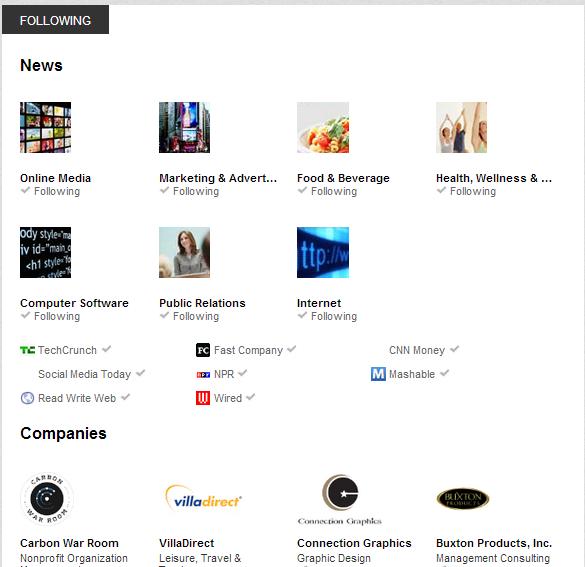The image features a white background with a mix of black and dark gray text. At the top, there's a black banner containing white text that reads "Following." Below this banner is a structured layout composed of four columns and two rows, listing various categories that the user is following. The categories include:

1. Online Media
2. Marketing and Advertising
3. Food and Beverage
4. Health, Wellness (text cuts off with ellipses)
5. Computer Software
6. Public Relations
7. Internet

The second row appears incomplete, featuring only three categories.

Interspersed within this layout are several recognizable websites also marked as being followed:
- TechCrunch
- Social Media Today
- ReadWriteWeb
- Fast Company
- NPR
- Wired
- CNN Money
- Mashable

Beneath this section is another header titled "Companies," under which several company logos are displayed. This segment features four columns, though only one row is fully visible, cut off abruptly. The companies listed include:

- Carbon
- War Room
- Villa Direct
- Connection Graphics
- Buxton Products Incorporated

Each company logo is accompanied by a brief subtitle that explains the nature or industry niche of the company.